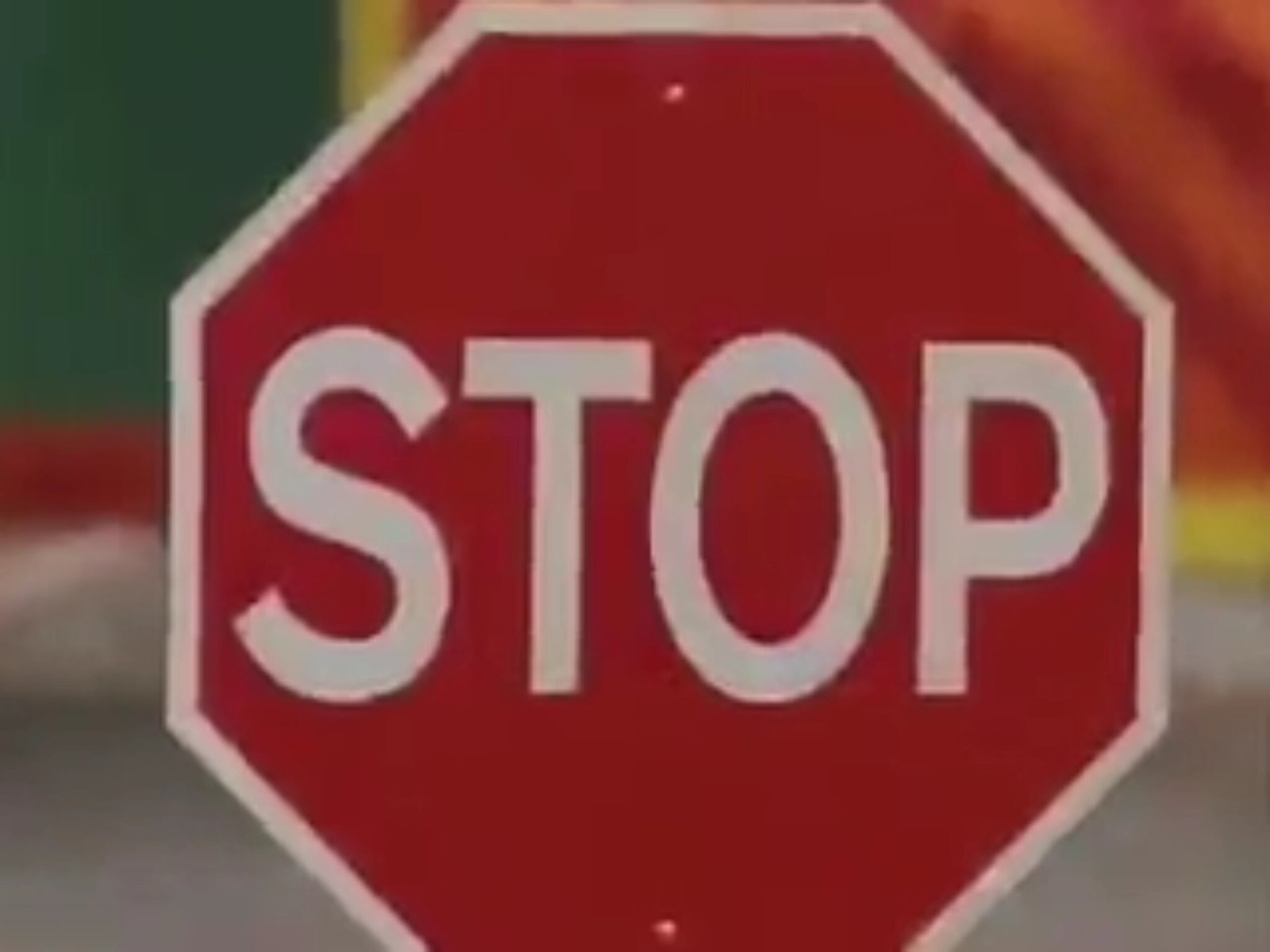This close-up photograph features an octagonal stop sign prominently in the center, vividly displaying its iconic red background with bold, white capital letters spelling "STOP." The sign is bordered by a thin white line, and there are two small rivets resembling white dots at the top and bottom. The background is heavily blurred, yet patches of color can be discerned, including a blotch of green and horizontal lines of yellow and red. Additional indistinct areas of reddish and yellow hues, along with light to dark gray tones, are scattered around the periphery. These colors suggest the presence of a wall or other surfaces, though the details remain indeterminate due to the photograph's focus on the stop sign. The bottom edge of the sign is slightly cut off, excluding the metal post that typically supports it.